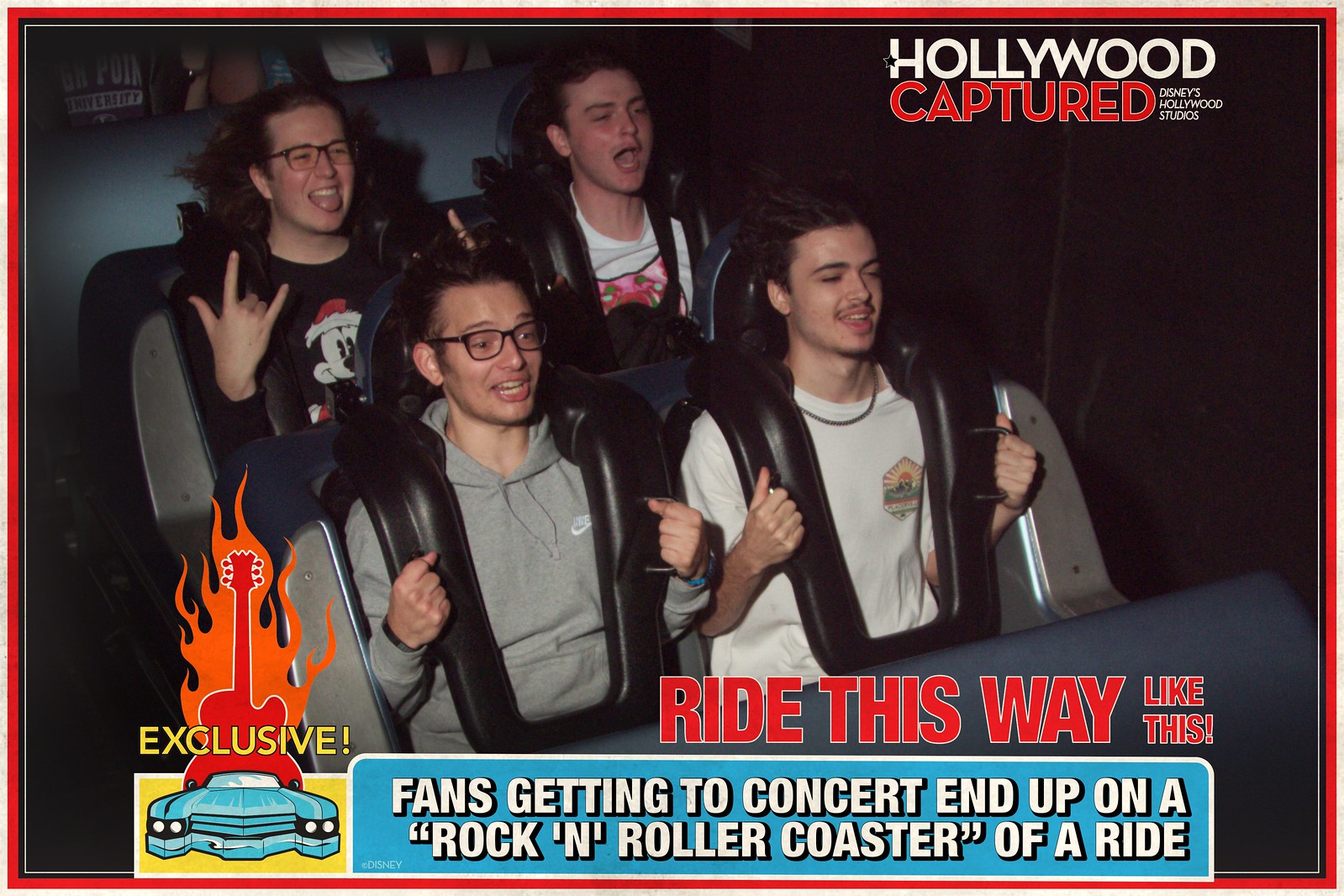The photograph, framed by a vibrant red border, captures the exhilarating moment of four individuals strapped into a roller coaster car. At the top right-hand corner, the words "Hollywood" in white font and "Captured" in red font signify the location: Disney’s Hollywood Studios. The image showcases the riders, all with dark brown or black hair flowing wildly, expressing sheer excitement. One rider prominently displays the "metal horns" hand gesture. The roller coaster car is framed by a black structure with silver seating and metal bars for safety. At the bottom right of the image, the red font reads "Ride This Way Like This," while a yellow box on the left side contains a blue catalog with a flaming guitar icon above it, exuding orange flames. Overlaid with the guitar is the word "Exclusive" in yellow. Adjacent to it, a blue box with white text announces, "Fans Getting to Concert End Up on a Rockin' Roller Coaster of a Ride."